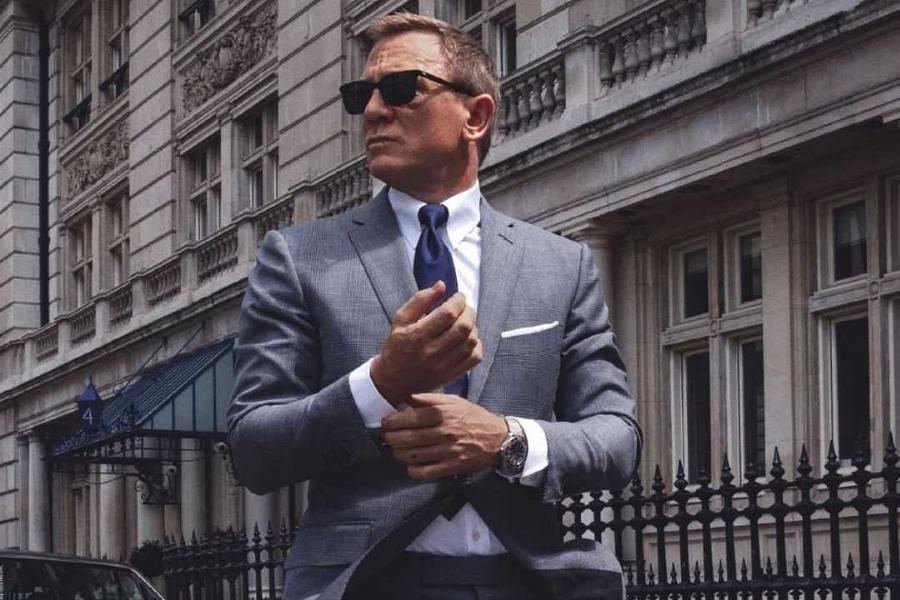This photograph captures a man striking a pose reminiscent of James Bond, particularly resembling the Daniel Craig incarnation of the character. He stands confidently in the daytime, wearing a well-tailored gray suit with a white shirt, a blue necktie, and black sunglasses. Short-haired and possibly bearing a few facial cuts, he exudes a tough yet sophisticated aura. The man is in the midst of adjusting his right cuff with his left hand, which also sports a silver watch. 

In the background, there are gray buildings adorned with ornate designs, columns, and wrought iron gates, suggesting a European urban setting. The presence of balconies, a series of windows, and architectural details further enhances the scene's elegance. Sunlight bathes the entire setting, creating sharp contrasts and highlighting the intricacy of both the man's attire and the backdrop. A car can just be seen peeking into the frame, reinforcing the impression that this could be a capture from an action-packed scene in a movie, possibly a James Bond film. The image is cropped to show him from the waist up, focusing on his expression and attire, adding to the sense of mystery and intrigue.